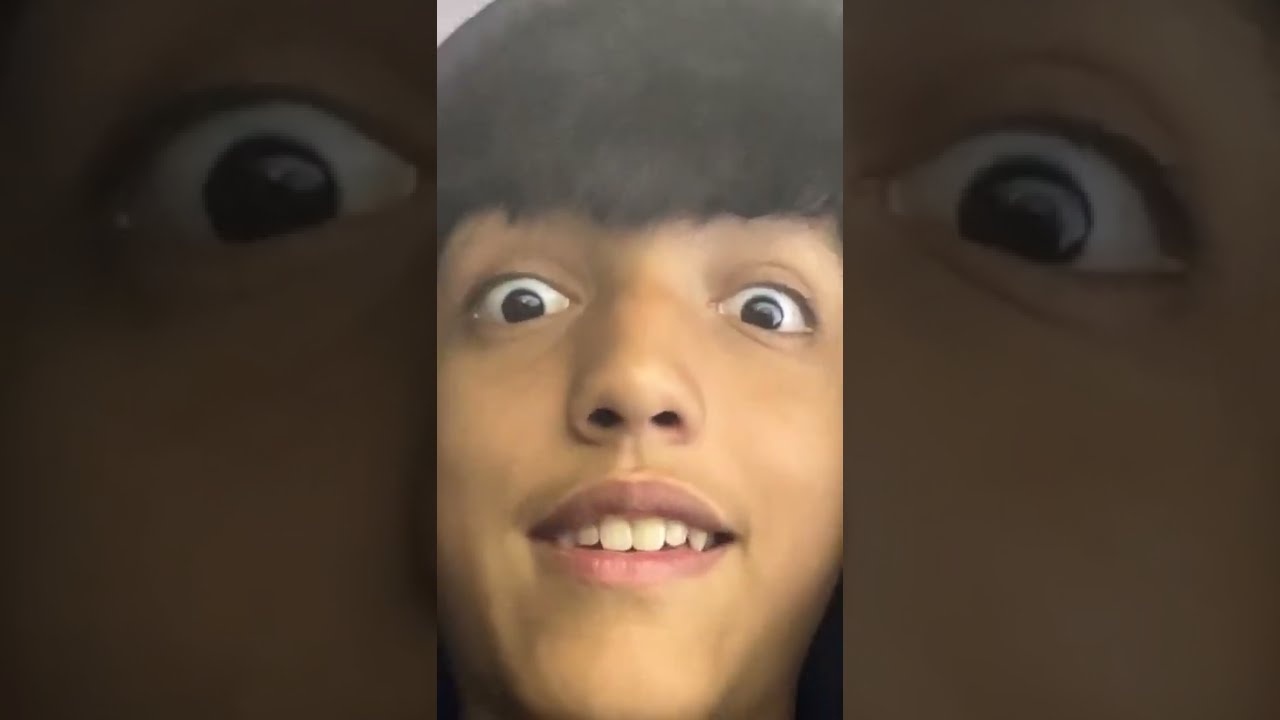This horizontal rectangular picture features a close-up, vertical rectangle at the center, showcasing the face of a boy who appears to be around 10 years old. His black hair falls as bangs just above his large, wide-open brown eyes, giving an impression of surprise or excitement. His mouth is open in a smile, revealing his top white teeth. The sides of his face are not visible, making it a narrow, focused shot of his facial features.

Flanking the central image on both sides are two larger vertical rectangles that create a background effect. The left rectangle is a highly zoomed-in close-up of the boy's right eye, while the right rectangle mirrors this with a close-up of his left eye. The lighting in these side rectangles is darker compared to the brighter central image, which has a hint of sunlight at the top and shadow towards the bottom underneath his chin.

The colors present in the image range from off-white and gray to black, brown, white, and pink. There is no text in the picture, and the style suggests it might be a selfie, possibly taken for a social media app like Instagram. The overall composition draws attention to the boy's expressive eyes and cheerful demeanor, complemented by the artistic background effect provided by the close-up eye images on either side.